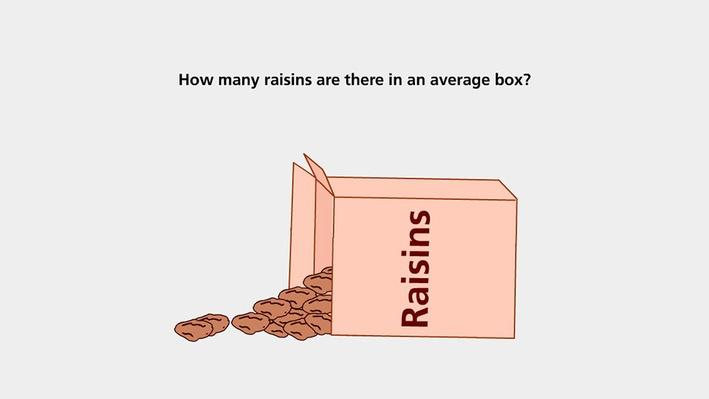The image depicts a pink cardboard box labeled "raisins" that is tipped over to its left, with brown raisins spilling out from its opening. The box occupies the center towards the bottom of the image, against a light gray background. Above the box, a caption asks, "How many raisins are there in an average box?" The text and design suggest it might be part of a trivia contest slide.